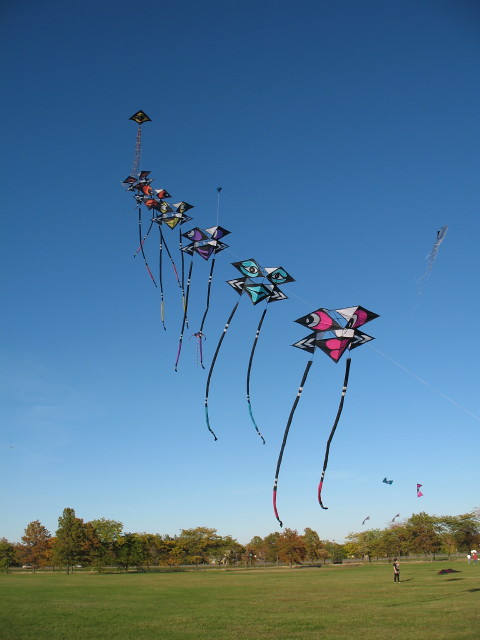This outdoor photograph captures a serene park scene dominated by an expansive, green lawn and scattered trees occupying the bottom fifth of the image. In this vibrant setting, one or two people are visible, appearing small amid the vast greenery. The striking, cloudless sky transitions from a light blue near the horizon to a darker, almost navy blue at the top, making up the remaining four-fifths of the portrait-oriented image. 

The sky is alive with five distinct kites arranged in a diagonal line stretching from the center-right towards the top left of the frame. These colorful kites—pink, teal, purple, yellow, and orange—each sport a pair of eye-like designs, giving them a whimsical, face-like appearance. Each kite is further adorned with two long tassels hanging from either side, swaying like legs as they catch the breeze. The lines controlling the kites are faintly visible, connecting them to unseen flyers on the ground. 

This playful arrangement of kites dominates the visual center of the photo, creating an enchanting juxtaposition against the undisturbed sky. Amidst this picturesque scene, the kites float effortlessly, framed by the tranquil park below and the gradient blue sky above, capturing a moment of simple, joyful recreation.